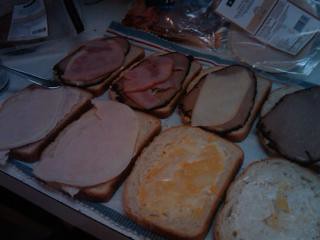A dimly lit photograph captures the preparation of several open-faced sandwiches on a white linoleum countertop. There are eight slices of bread arranged in two rows and four columns, each with various toppings. The four bottom slices feature either turkey or ham, with one showing a spread that resembles mayonnaise or cheese. The top slices of bread appear to have either roast beef or pastrami, with one also displaying a slice of melted cheese. In the top corners of the image, two packages of lunch meat can be seen, one with a visible white label and UPC code. A knife or spoon peeks out from under one of the lower-left sandwiches. The bread and toppings rest on a white towel with blue and red stripes, adding a subtle pattern to the composition. The dim lighting creates a moody atmosphere, making the details of the meat and spreads somewhat harder to distinguish.